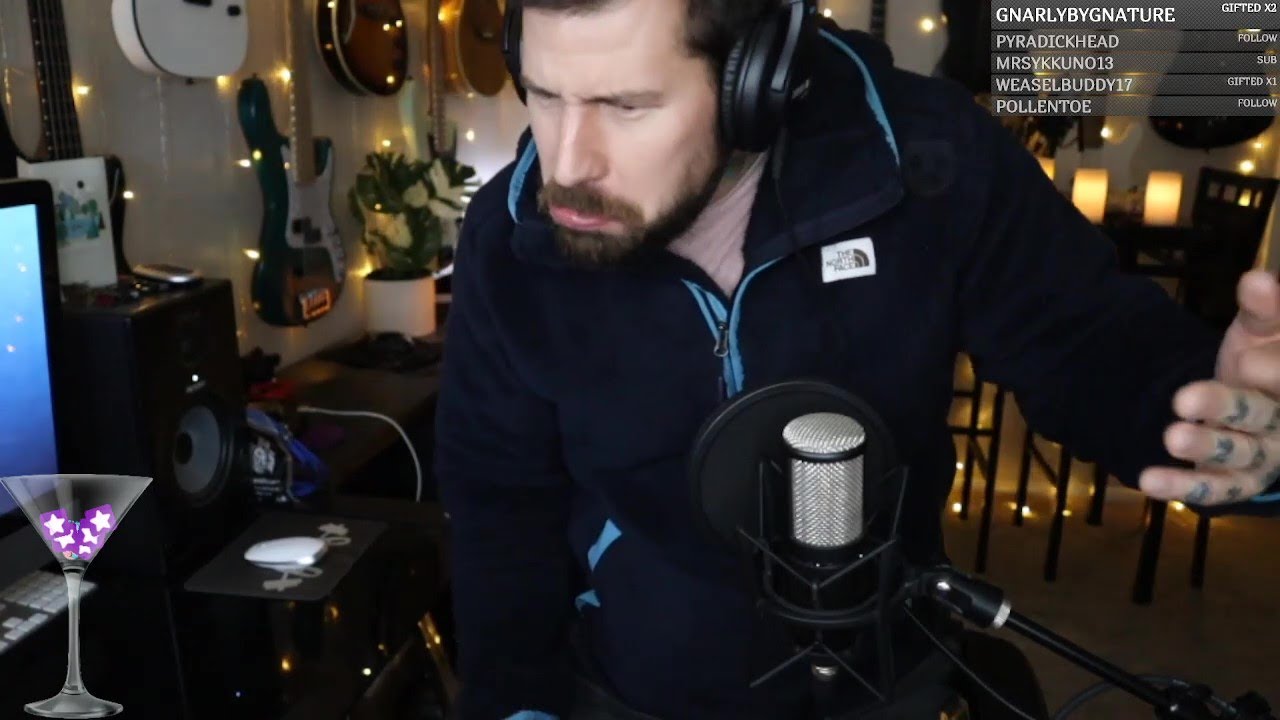A detailed caption for the image:

In this vibrant screenshot taken from a laptop, we see a light-skinned male participating in what appears to be a podcast, live interview, or live performance. The image prominently displays the upper right-hand corner of the screen, featuring the text "GNARLY BY NATURE," followed by "gifted x2,” "pirate dickhead," "follow," "Mrs. YKKUNO13 sub," "weasel buddy 17 gifted x1," and "paw and toe follow." 

At the bottom left-hand corner, there's a digital icon of a martini glass adorned with purple and white stars. The main subject, centered in the frame, has a brown beard and mustache, and is wearing heavy earphones. Positioned in front of them is a large microphone with a cover. They are dressed in a fluffy blue jacket with matching trim. The person's left hand is raised to the right side of the image, revealing tattoos across their fingers. 

In the background, the upper left corner reveals a collection of guitars hanging on the wall, adding a musical theme to the setting.